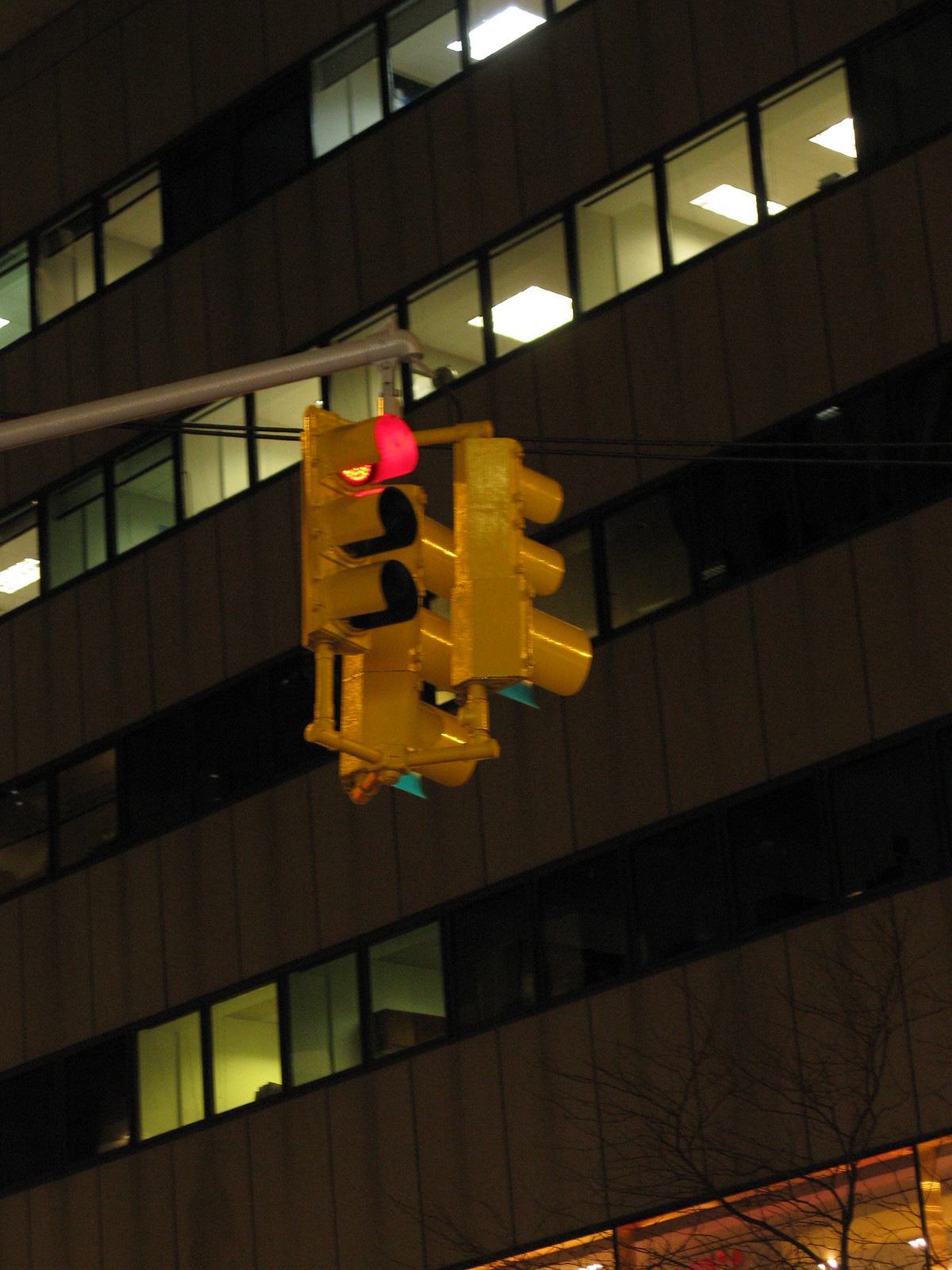In this semi-close-up nighttime photo, we see a traffic light mounted on a beige pole, overhanging what appears to be a road, though the roadway itself is cropped out. The traffic light fixture is yellowish-orange and comprises three sections displaying red, yellow, and green lights. The light facing the camera shows a lit red signal, while the other two lights, angled away from the camera, reflect green. The backdrop features a multi-story commercial or office building, with four visible floors lit by a mix of on and off fluorescent lights. Additionally, tree branches without leaves are visible in the bottom portion of the frame, adding more context to the scene. Despite the moderate photo quality, the details of the illuminated windows and the various lights are clear.